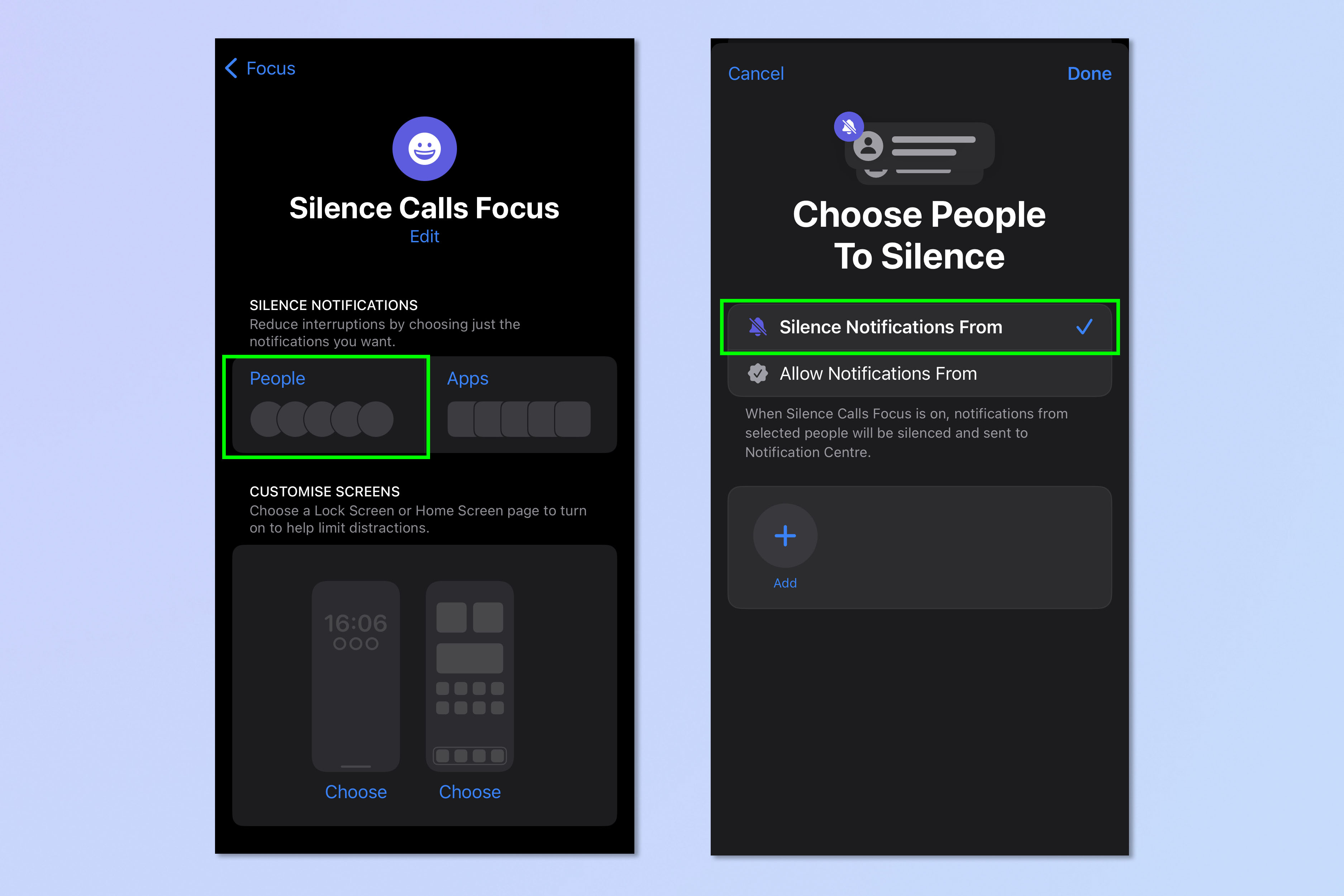The image features two mobile screenshots displayed against a light pastel blue background. 

**First Screenshot**:
- The background is black.
- At the top left, there is blue text that reads "Focus" with a blue arrowhead pointing left.
- Centrally positioned at the top, there is a violet-blue circle containing a white smiley face.
- Below the circle, the text "Silence calls & notifications" is displayed in bold white font.
- In a smaller blue font centered underneath, the word "Edit" is visible.
- Towards the left, the white capitalized text reads "Silence notifications."
- Beneath this, in gray text, it states: "Reduce interruptions by choosing just the notifications you want."
- Further below, the blue text "People" appears next to several overlapping circles, intended for adding different contacts. This section is highlighted with a lime green rectangular border.
- To the right, there is an overlay of several blank app icons. At the upper left of this section, the blue text reads "Apps".
- Below this, the capitalized white text "Customized screens" is followed by the gray text: "Choose a lock screen or home screen page to turn on to help limit distractions."

**Second Screenshot**:
- The background is also black.
- The header "Choose people to silence" is displayed in white at the center.
- Below this, there is a medium gray background area.
- On the left side of this area, there is a violet notification icon with a slash through the middle, indicating silencing.
- To the right of the icon, the white text reads: "Silent notifications from".
- A blue checkmark towards the right is also visible, highlighting this section with a lime green rectangular border indicating that it is selected.